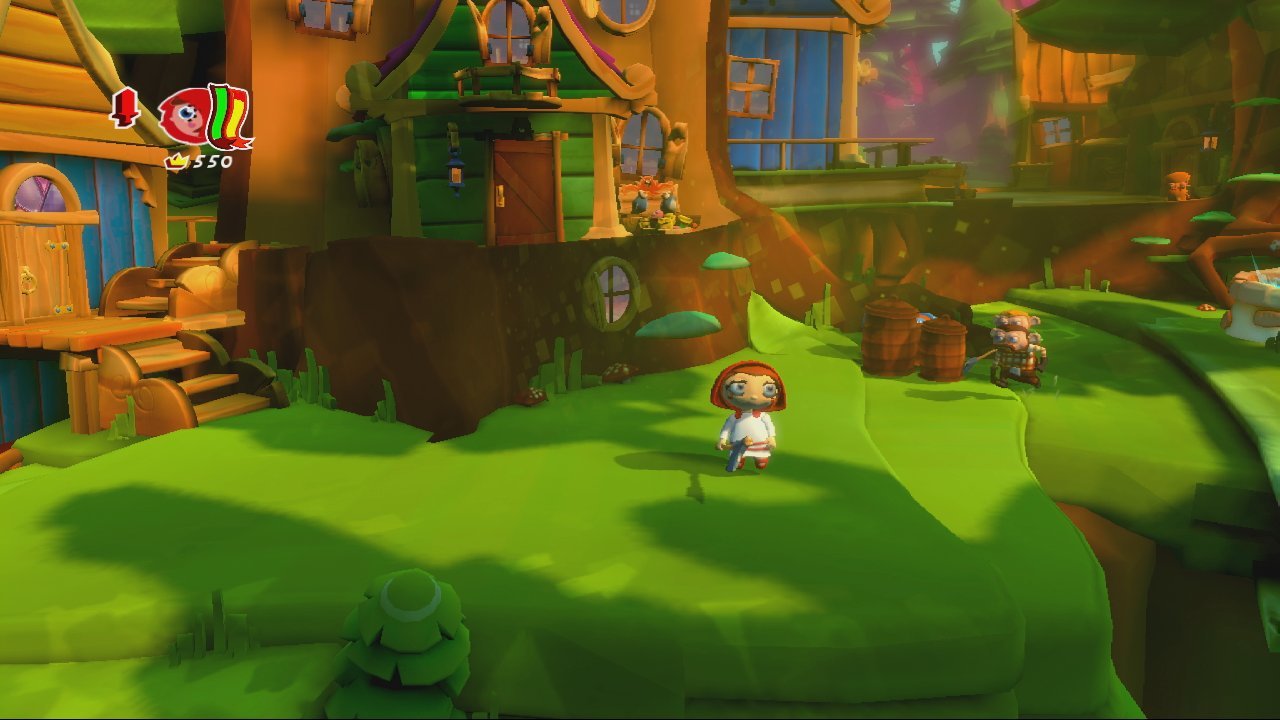This image is a detailed screenshot from a modern animated video game designed for children. The scene shows a vibrant, cartoonish environment with several whimsical tree houses in the background. The houses are perched on tree trunks with brown wooden doors and colorful windows in hues of blue, purple, and green. One house features a balcony and is connected by steps to another standalone house. 

In the foreground, a meticulously cut green lawn transitions sharply into a brown cliff edge on the right. Dominating the scene is a small cartoon character, seemingly female, with auburn hair, large round eyes, and light skin. She wears a white dress or tunic, possibly with a belt, and stands near two wooden barrels. Beside her, a smaller character, potentially an older male, stands partially obscured. 

To the left of the scene is a superimposed logo, roundish in shape with reddish-pink, yellow, and green accents, and featuring a partial face with one eye. Below this logo, the number "550" is prominently displayed, likely indicating a score or level identifier.